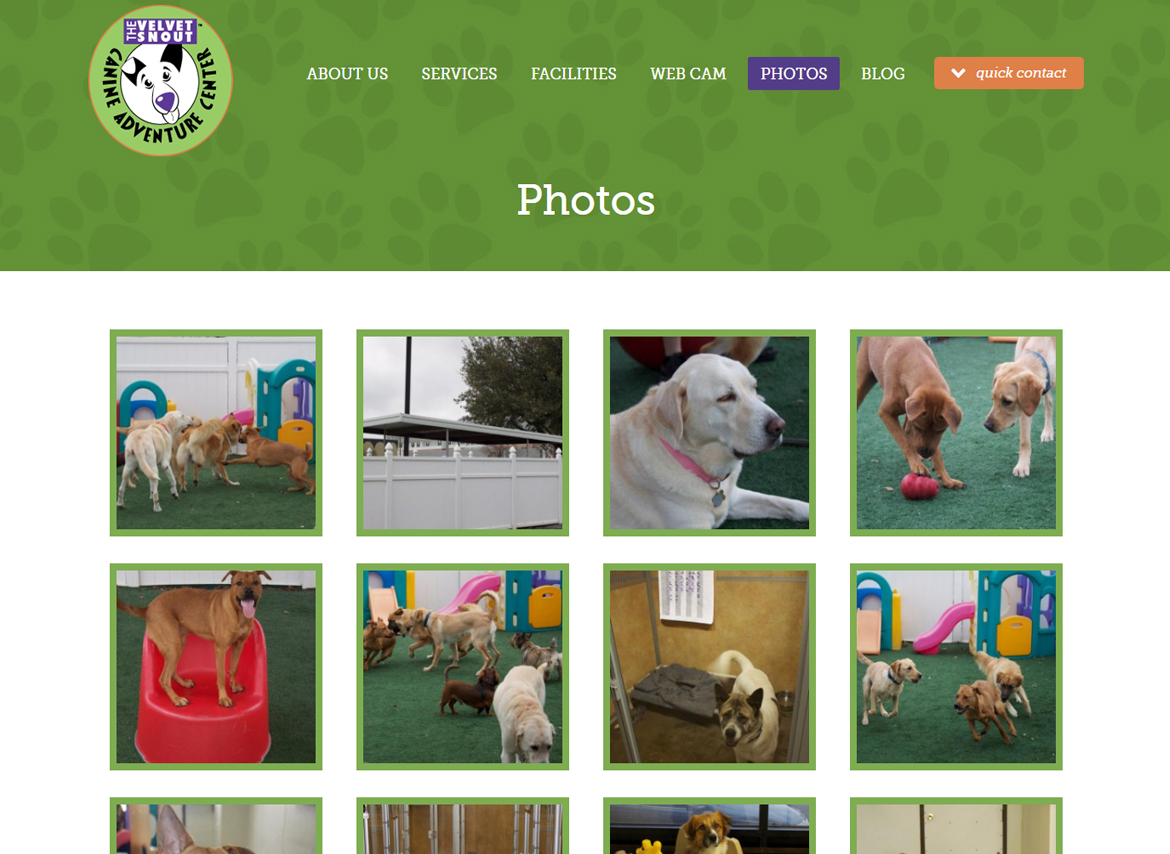This screenshot captures the homepage of a website for a dog daycare center named "The Velvet Snout Canine Adventure Center." At the top left corner, the logo features a whimsical illustration of a dog with its tongue out, enclosed within a circle. The logo prominently displays the center's name, "The Velvet Snout," atop a purple background. Encircling the bottom half of the logo is the text "Canine Adventure Center."

The navigation bar beneath the logo includes several buttons: About Us, Services, Facilities, Webcam, Photos (currently selected), Blog, and a Quick Contact drop-down menu.

The main content section showcases a series of photos depicting dogs in various playful settings. The top left photo features three dogs joyfully interacting in a well-equipped dog playground. To the right, there's an image of a facility gate, followed by a German Shepherd. Next, an adorable puppy is seen playing with a tomato, accompanied by another dog.

In the second row, the leftmost image shows a dog standing on a plastic structure reminiscent of a bath. Adjacent to this, multiple dogs are engaging in play on the playground. Further right, there's a cozy dog bedroom with a little bed occupied by what seems to be a Husky. The final image in the row shows three more dogs frolicking on the playground.

The bottom of the screenshot partially displays additional dog photos, hinting at more delightful imagery below the visible portion.